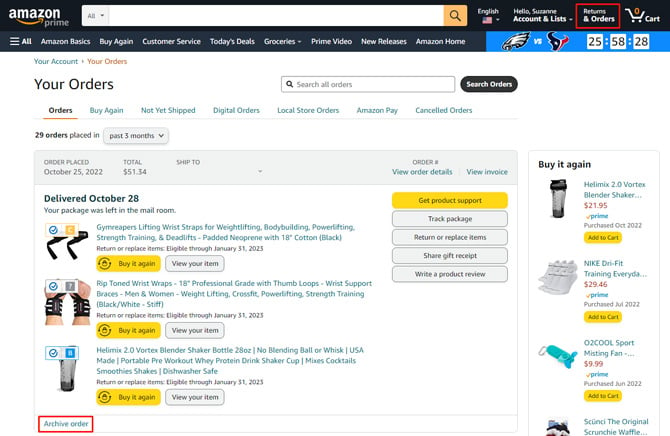The image displays the homepage of the Amazon website. In the top-left corner, there is an Amazon Prime logo. A black banner spans the top of the page, featuring a search box. To the left of the search box, there is a drop-down menu labeled "All," and to its right, a small orange box with a magnifying glass icon signifying search. Further to the right, the site language, "English," is displayed alongside an American flag. The text "Hello, Suzanne" appears, indicating the user is logged in. Options to access "Account & Lists" are next, followed by "Returns & Orders," which is highlighted with a red box. Nearby, there is an orange zero in the shopping cart icon.

Below the black banner, there are several categories listed: All, Amazon Basics, Buy Again, Customer Service, Today's Deals, Groceries, Prime Video, New Releases, and Amazon Home.

To the right of these categories, there is a blue rectangular box displaying a banner for an upcoming football game, presumably between the Philadelphia Eagles and another team, with a countdown timer showing "25:58:28," indicating the game starts in 25 hours, 58 minutes, and 28 seconds.

Further down, there is a section titled "Your Orders," displaying an overview of recent purchase activity. It notes that 29 orders have been placed in the past three months. One specific order is detailed, placed on October 25, 2022, totaling $51.34, and delivered on October 28. The delivery note specifies that the package was left in the mailroom. Items in this order include Jim Reapers lifting wrist straps for weightlifting, bodybuilding, powerlifting, strength training, and deadlifts, Riptone wrist wraps, and a Helamix 2.0 Vortex blender shaker bottle.